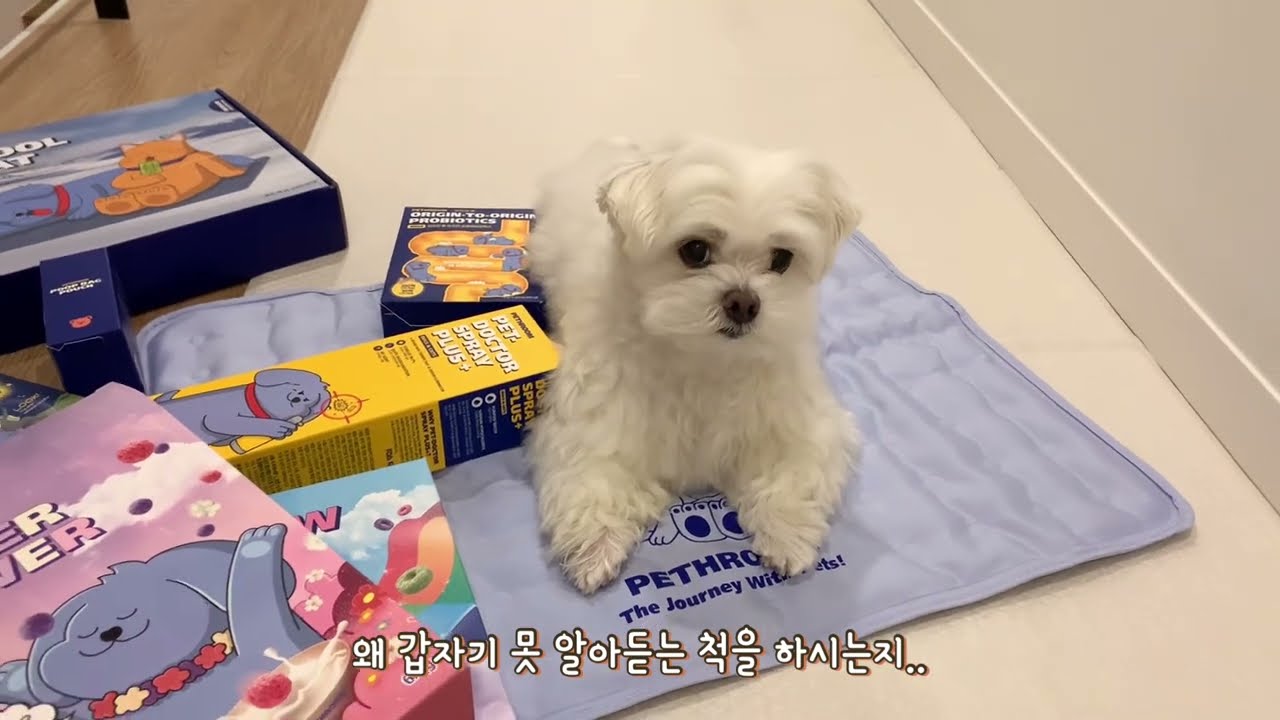In the image, a small white puppy, possibly a poodle, is sitting on a light purple blanket laid over a blue pet rug. The puppy, with its black eyes and nose, is positioned right in the center, resting on its forepaws. Surrounding the dog, primarily to its left and on the edge of the rug, are several boxes featuring cartoon animals. Notably, one box near the dog is yellow with a blue dog and white text, labeled Pet Doctor Spray Plus. Behind it, there's a blue box, and in front of that, a pink and blue box stacked together. Further left on the hardwood floor, another blue box can be seen, also decorated with cartoon imagery. The background includes a white wall with baseboard trim on the right and a brown hardwood floor leading up to the dog. A strip of carpet runs along the left side of the image, and at the top left, part of what appears to be a stand is visible. Along the bottom center of the image, there's text in Asian characters, possibly Japanese or Korean, although partially obscured.